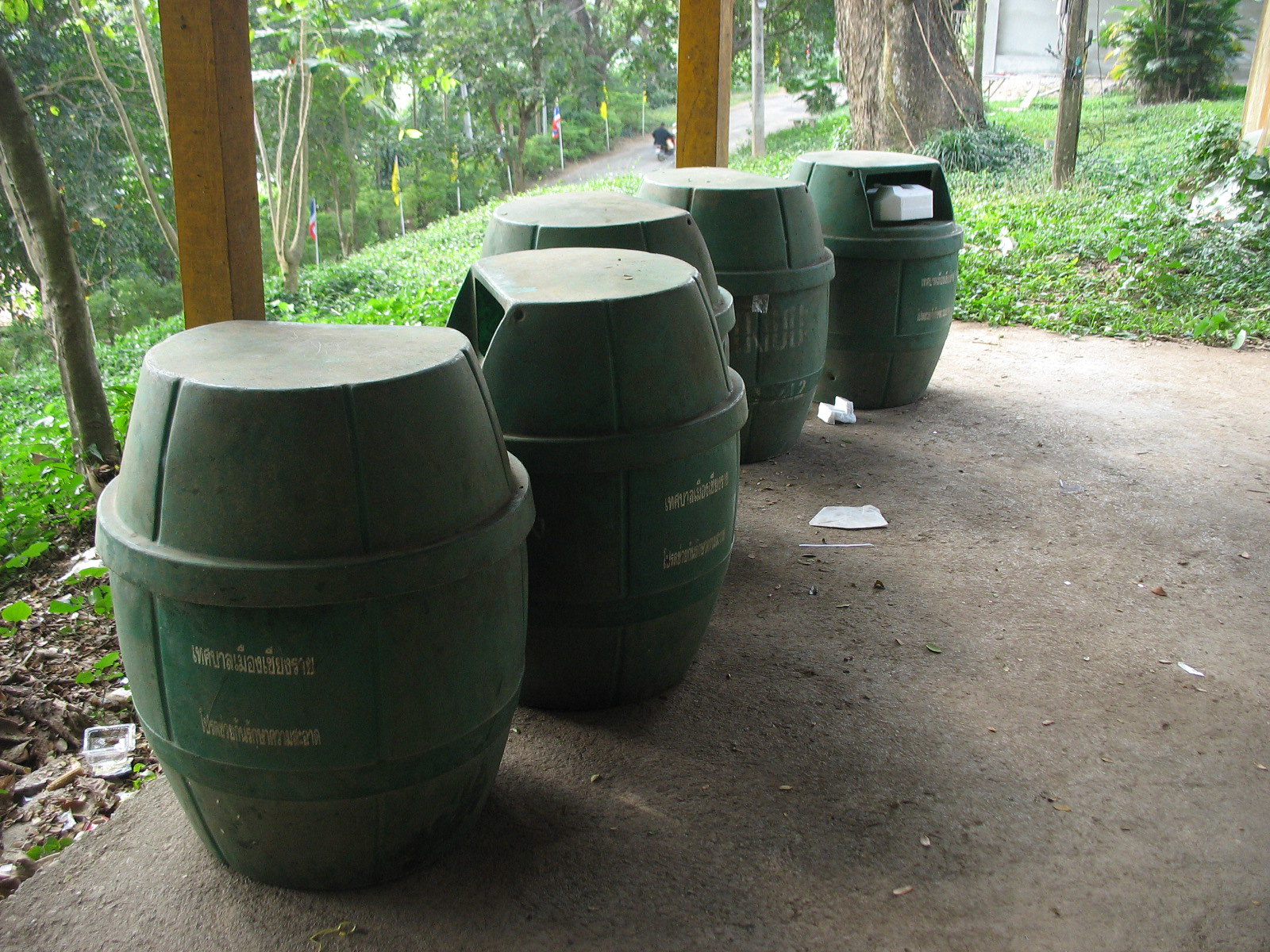The image depicts five green, barrel-shaped plastic bins, likely recycling bins, positioned on a concrete porch or floor. The bins are arranged facing different directions, and one of them contains a white cardboard box. Scattered on the ground around the bins is some visible debris, indicating that not all garbage made it into the bins. Nearby are two vertical, yellowish wooden beams, possibly part of a structure like an awning or gazebo, though the roof is not visible. The background reveals a lush, forested area with various trees and foliage. To the left, a path lined with flags runs through the scene, and a person riding a bicycle or motorcycle can be seen on this path, adding a sense of life and activity to the wooded setting.